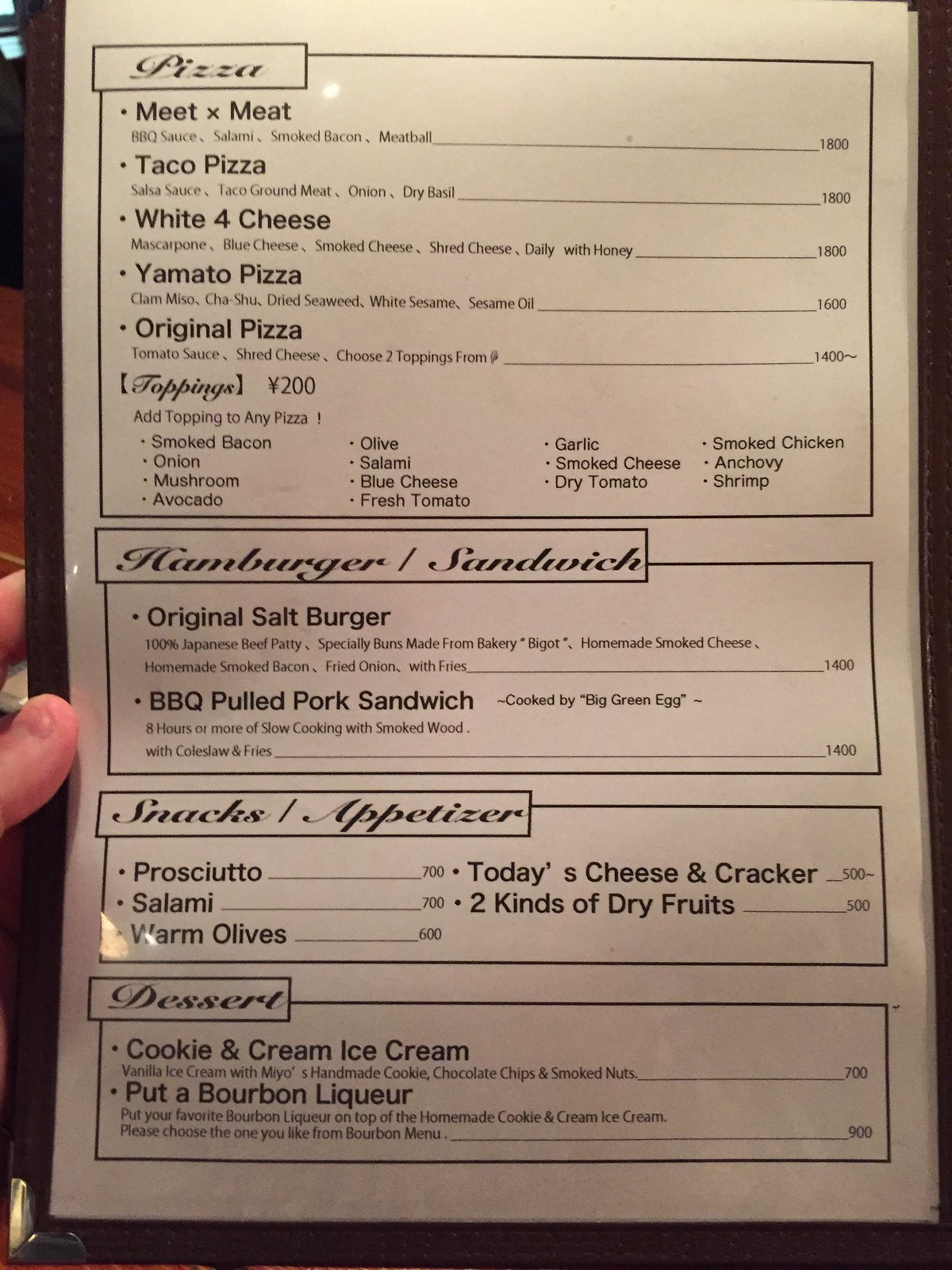The photograph captures a menu held in portrait orientation, showcasing a detailed array of food items with clear black text on a white background, encased in plastic which causes light glare at several points. The menu features a distinct black border and is being held by someone's thumb and forefinger, visible on the left side.

At the top, a black-outlined rectangle highlights the section titled "Pizza" in script. Underneath, various pizza options are listed:

- **Meat times Meat Pizza**: ¥1,800
- **Taco Pizza**: ¥1,800
- **White Four Cheese Pizza**: ¥1,800
- **Yamato Pizza**: ¥1,600
- **Original Pizza**: ¥1,400

Additionally, there is a list of extra toppings available for ¥200 each, including smoked bacon, onion, mushroom, avocado, olive, salami, blue cheese, fresh tomato, garlic, smoked cheese, dried tomatoes, smoked chicken, anchovy, and shrimp.

The next section, titled "Hamburger/Sandwich" in script, lists:

- **Original Salt Burger**: ¥1,400
- **Barbecue Pulled Pork Sandwich**: ¥1,400

Following this, the "Snacks/Appetizer" section includes:

- **Prosciutto**: ¥700
- **Salami**: ¥700
- **Warm Olives**: ¥600
- **Today's Cheese and Cracker**: ¥500
- **Two Kinds of Dry Fruit**: ¥500

At the bottom, the "Dessert" panel offers:

- **Cookie and Cream Ice Cream**: ¥700
- **Pudding Bourbon Liquor**: ¥900

This comprehensive menu provides a broad selection of appetizing options, meticulously organized into distinct categories for a clear and pleasant reading experience.